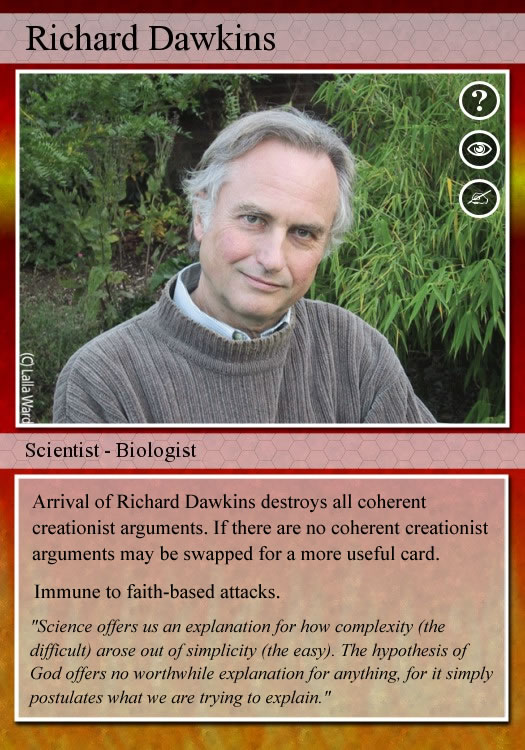This is an image of a mock playing card featuring Richard Dawkins. At the top of the card, "Richard Dawkins" is written in bold, black text. Just below the text is a photograph of an older man, identified as Dawkins, who is smiling and looking directly at the camera. He is dressed in a gray turtleneck sweater over a colored or white shirt. The background of the photograph contains plants and bushes. Towards the upper right corner of the photograph, there are three symbols: a question mark, an eyeball, and a hand holding a pen.

Below Dawkins' photograph, the text "scientist, biologist" appears in black. Further down the card, a separate text box states, "Arrival of Richard Dawkins destroys all coherent creationist arguments. If there are no coherent creationist arguments, maybe swap for a more useful card. Immune to faith-based attacks."

Additionally, the card features a quote from Dawkins: "Science offers us an explanation for how complexity, the difficult, arose out of simplicity, the easy. The hypothesis of God offers no worthwhile explanation for anything, for it simply postulates what we are trying to explain."

The card’s background showcases a gradient that transitions from orange at the bottom to a redder hue towards the top, intersected by a yellow line.